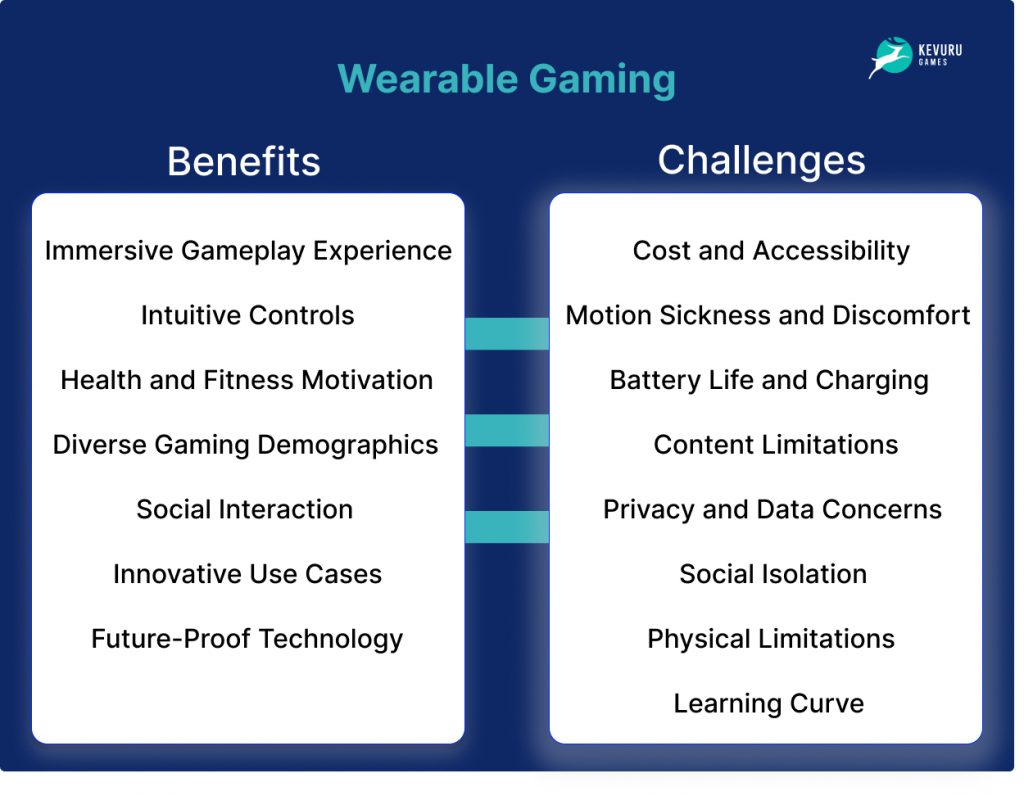The infographic features a dark blue background and prominently displays the title "Wearable Gaming" in light blue font at the top. In the upper right corner, there's the logo of Kevuru Games, spelled K-E-V-U-R-U, which includes an emblem of a deer leaping in front of what resembles a moon. Below the title, the infographic is divided into two white rounded text boxes. The left box is labeled "Benefits" and lists points such as Immersive Gameplay Experience, Intuitive Controls, Health and Fitness Motivation, Diverse Gaming Demographics, Social Interaction, Innovative Use Cases, and Future-Proof Technology. The right box is labeled "Challenges" and lists issues like Cost and Accessibility, Motion Sickness and Discomfort, Battery Life and Charging, Content Limitations, Privacy and Data Concerns, Social Isolation, Physical Limitations, and the Learning Curve. Connecting the two sections are three light blue, almost turquoise, lines.